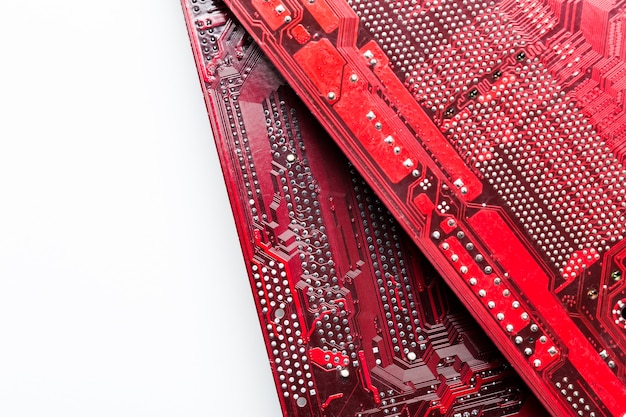The image shows a close-up of two red circuit boards positioned diagonally and stacked on top of each other, primarily occupying the center and right side of the frame. The upper board, which is brighter red, features several rows and columns of tiny white dots clustered together, adding intricate detail to its surface. In contrast, the lower board is a darker shade of red and is adorned with small silver metallic balls, possibly solder points, near the clustered white dots on the upper board. The left third of the image is empty, filled with white space that fades into a faint grayish hue, creating a stark contrast to the intricate and vibrant elements of the circuit boards. No text or additional descriptive elements are present in the image.